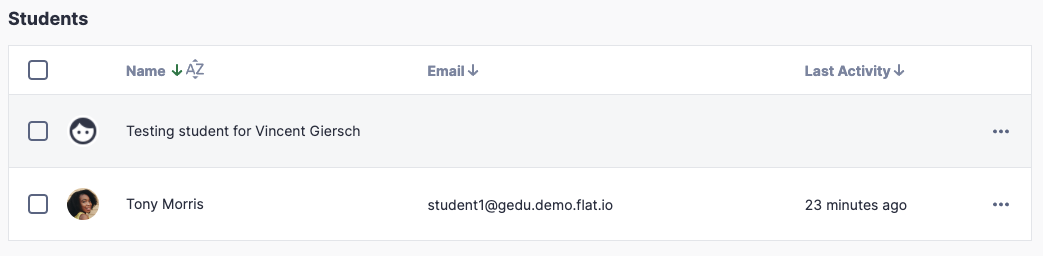The image displays a minimalist table designed to track student information, specifically their names, email addresses, and recent activity timelines. The table includes two entries: one for Vincent Gersh and another for Sonny Morris. Sonny Morris' email is listed as student1.demo@flat.io, and his last activity was recorded 23 minutes ago. The background of the image is a clean, unobtrusive white, ensuring that the focus remains on the table's content. There are no additional elements or details present in the image, highlighting its simplicity and clarity.